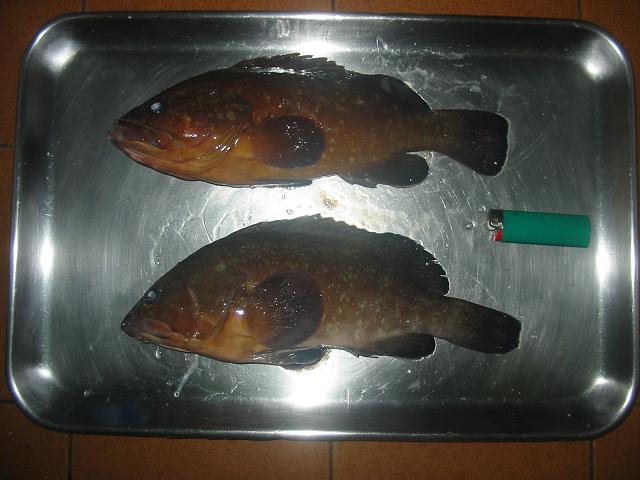This detailed color photograph, captured in a landscape orientation, presents a top-down view of two dead fish laid out in a rectangular, silver-colored metal baking pan with rounded corners. The pan, which rests on a counter covered with brown tiles, contains the fish placed side by side with their bodies positioned on their sides. The fish are light brown with dark fins and pointed mouths, and they are medium in size — not particularly large. A notable element in the composition is an aqua-colored cigarette lighter with a red button, situated between the fish on the right side of the pan, presumably to provide scale. The overall scene hints at preparations for a meal, although the unusual inclusion of the lighter adds an element of ambiguity or potential symbolism.